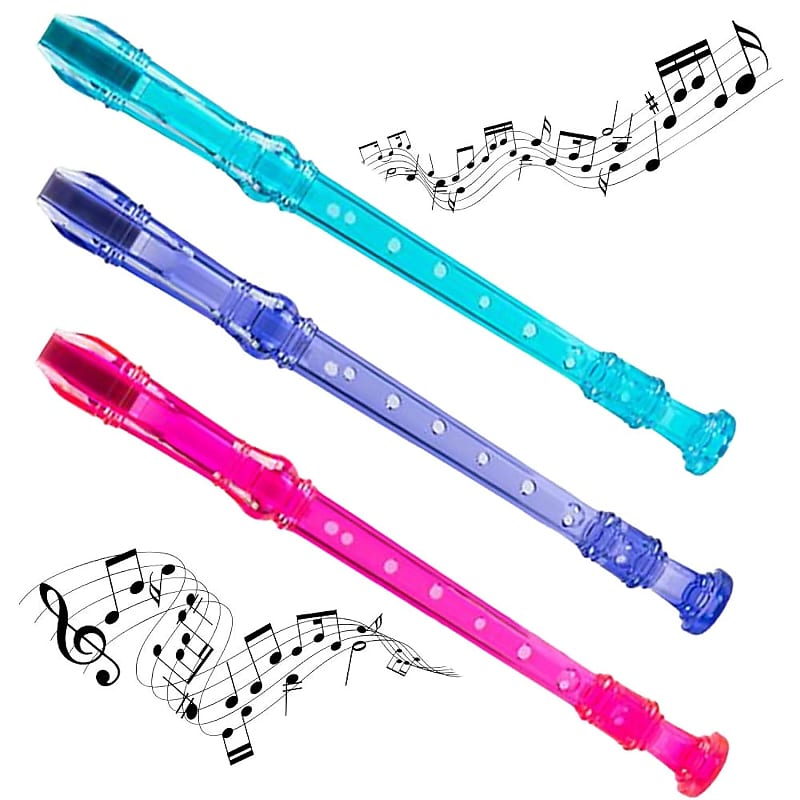The image features three translucent plastic recorders arranged diagonally against a white background. The recorders are identical in size and shape, but in different vibrant colors: an aqua blue recorder at the top, a lavender one in the middle, and a hot pink one at the bottom. Each recorder has evenly spaced finger holes, a rounded mouthpiece end, and a tapered end. At the upper right corner of the image, there is a strand of musical notes flowing in a wavy pattern from left to right, while at the bottom left, another strand of musical notes spirals in a wavy fashion, fading out toward the edges. The notes in both strands are black.